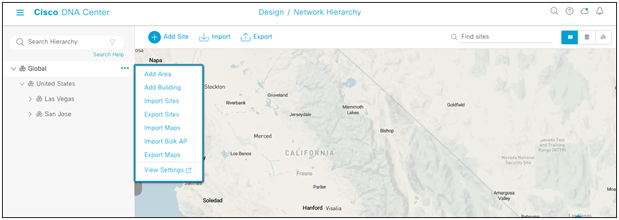Screenshot Description:

The screenshot showcases a user interface from Cisco DNA Center, designed with a light-colored, pastel aesthetic, incorporating hues of light green and very light blue. At the top of the interface, the word "DNA" and the title "Cisco DNA Center" are prominently displayed in turquoise. Directly below this, there are three horizontal lines representing the menu, along with options labeled "Design/Network Hierarchy," "Share," "Question," and "Alarm."

Further down, a search button followed by an "Add Site" button is visible, providing the option to click and choose various sites. This section also includes functionality for importing and exporting data, along with a search bar. Beneath the search bar, the hierarchical structure starts with "Global" at the top, followed by "United States," "Las Vegas," and "San Jose." A distinct black border outlines the map.

The map within the interface highlights the state of California, with detailed geographical features like water bodies.